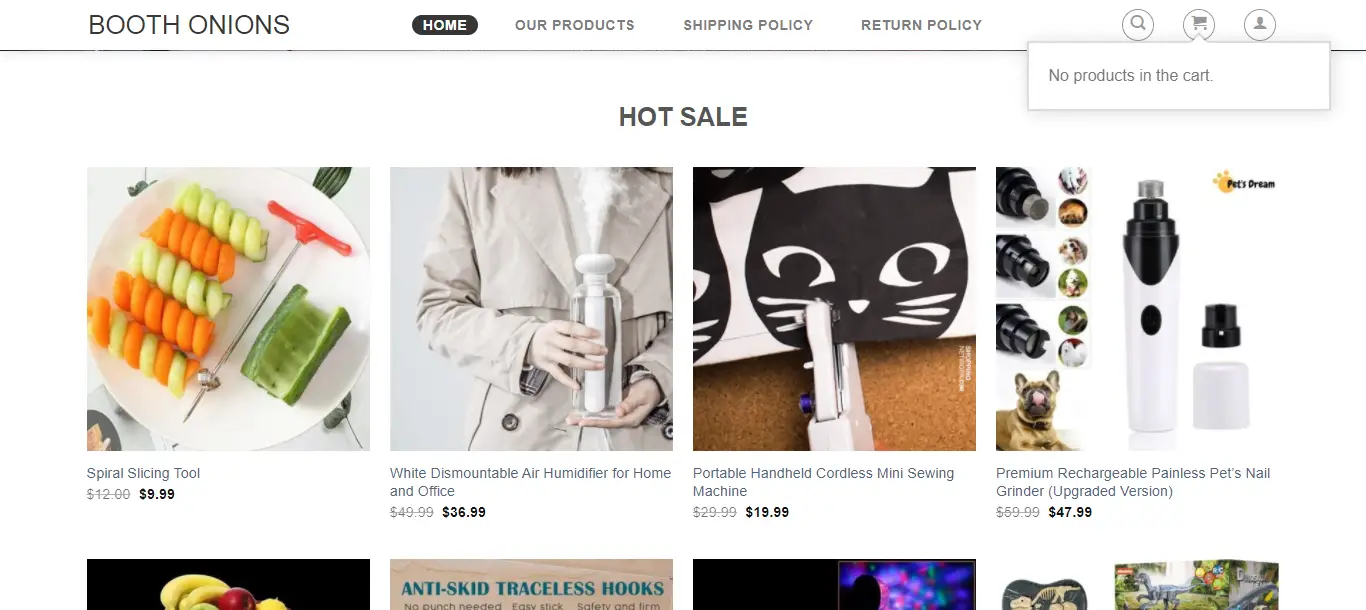A computer screen displaying a shopping website is shown with a white background. At the top of the screen, a thin black or grey line runs horizontally, separating the navigation menu from the main content. Above this line, the website's navigation is displayed, featuring "Booth Onions" in bold black capital letters on the left. Centrally positioned above the line are navigation links for "Home," "Our Products," "Shipping Policy," and "Return Policy." On the right, three circular icons are visible: a magnifying glass for search, a shopping cart, and a person icon for user account. The mouse cursor hovers over the shopping cart icon, triggering a pop-up message that reads "No products in the cart."

Below the navigation menu, bold grey capital letters announce a "HOT SALE." Four images of various products are visible, with a partial view of an additional four images beneath them. The showcased products include a spiral slicing tool, an air humidifier, a cordless sewing machine, and a painless pet nail grinder, along with their respective prices. The screen captures a detailed snapshot of the online shopping experience, highlighting both the site’s interface and a selection of featured items.